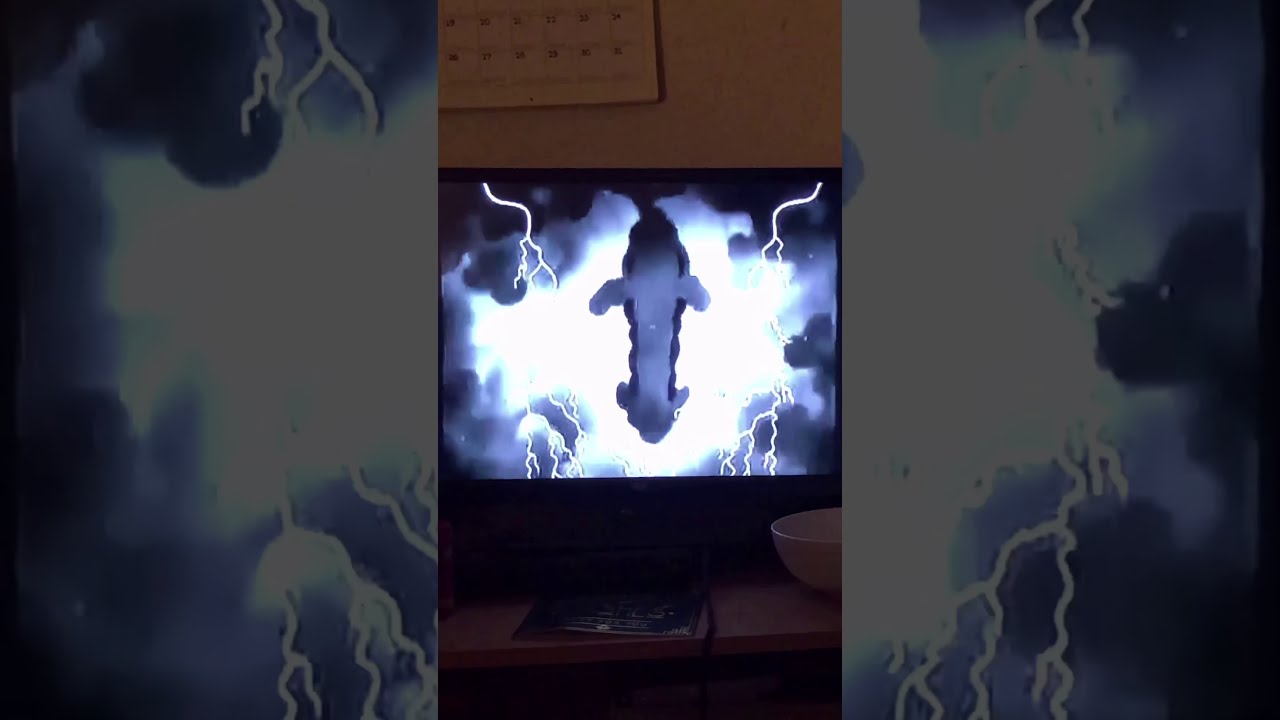In this vertically oriented cell phone image, a TV screen prominently occupies the center, flanked by larger, blurred sections of the scene on either side. The TV is perched on a brown wooden table, with a white bowl to its right and a dark-colored piece of paper or magazine positioned in front. Above the TV, a beige wall holds the bottom lines of a calendar, visible in the upper center-left area.

The TV screen displays a vivid, somewhat cartoonish image of storm clouds. Dark, purplish clouds frame the screen's corners, with jagged white lightning zigzags extending from multiple points. The center of the screen is dominated by a bright white light, making the clouds appear as if they are glowing. Amidst this brightness, a dark bluish-black shape, reminiscent of an airplane fuselage with short wings, emerges from the clouds. The surreal, stormy atmosphere captured on the TV contrasts with the mundane living room elements, encapsulating a moment where the extraordinary meets the everyday.